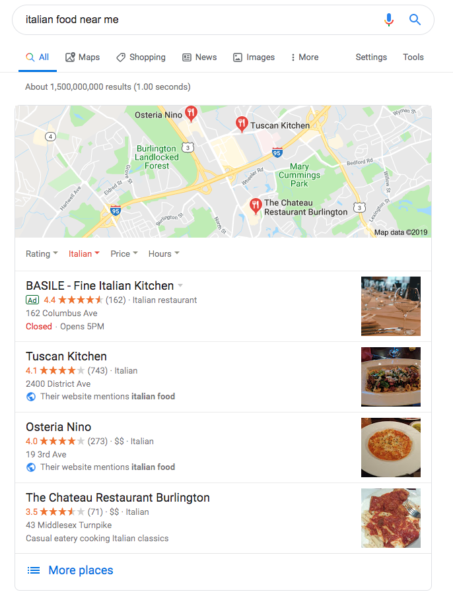The image displays a Google search results page for the query "Italian food near me." At the top, there's a long, oval-shaped search bar with a light gray border. Inside the search bar, the text "Italian food near me" is typed in black. Towards the right inside the search bar, there's a microphone icon followed by a blue magnifying glass icon.

Below the search bar, a navigation menu contains several clickable tabs. The "All" tab is highlighted in blue with a multicolored magnifying glass icon to its left and is underlined by a bold blue line indicating it's selected. Other tabs labeled in gray include "Maps," "Shopping," "News," "Images," and a "More" option represented by three dots. Further to the right are "Settings" and "Tools."

Beneath the navigation menu, small gray text shows the total results as "About 1,500,000,000 results (1.00 seconds)." A map section featuring red map pins follows, highlighting locations such as "Ostiera Nino" at the top-left, "Tuscan Kitchen" in the middle-right, and "The Chateau Restaurant of Burlington" towards the bottom.

Further down, the page transitions into a white section with four distinct drop-down menus labeled "Rating," "Italian," "Price," and "Hours." The "Italian" menu is selected, indicated by its red color. The first search listing is for "BASILE - Fine Italian Kitchen" in black text, accompanied by a gray arrowhead for a drop-down menu. To the right of this listing, a green outlined rectangle with the word "Ad" in green signifies a sponsored result. Adjacent to this, an orange text displays a rating of "4.4," with a corresponding 4.4 out of 5 stars filled in orange.